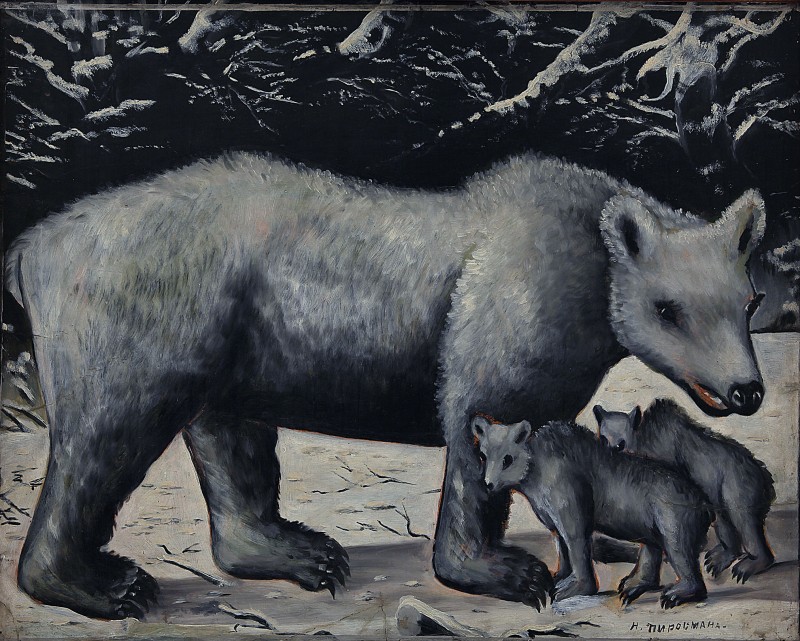This is a captivating painting done predominantly in shades of black, white, and gray, with intentional accents of red. The central focus is a large, bear-like creature occupying most of the canvas. This creature, which walks on four legs, has a hump above its front shoulders and a short tail. Its head is lowered, revealing a flared nose reminiscent of a deer's, and an open mouth with visible red and white teeth. The bear's figure is detailed with thick, curved claws on its paws. 

Standing on a barren, light-colored ground, likely white or cream, the main bear is accompanied by two smaller cubs positioned beneath its neck and oriented to the left. Both the adult bear and one of the cubs have subtle red accents: the adult's mouth and the cub's ear and leg borders. The background conveys a sense of mystery with irregular shapes resembling tree branches or perhaps animal skeletons amidst dark and gray shades, giving the upper half an almost cavernous feel.

The painting's stark and detailed composition captures a sense of the wild and the unknown. In the lower right corner, it is signed, though the signature is somewhat illegible, deciphered only partially with elements like H, T-I-M-P-O-L-M-A-H-A. This enigmatic signature complements the overall mystique of the artwork.